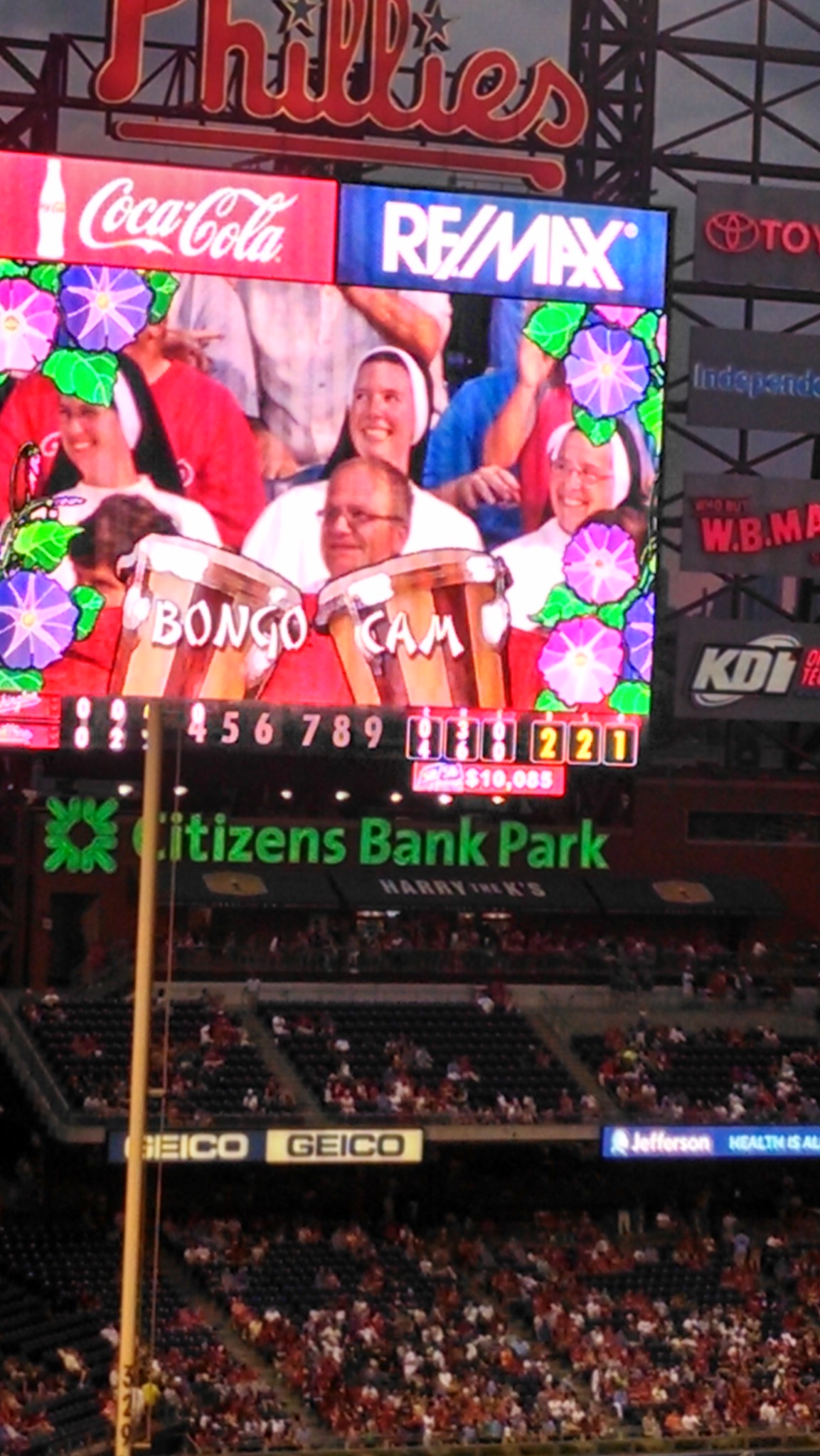The photograph captures a vibrant scene at Citizens Bank Park during a Phillies baseball game. The image, oriented in portrait mode, showcases the stadium's stands filled with enthusiastic fans. At the very top, in bold red letters, "Phillies" is prominently displayed, each "i" adorned with a star. Directly below, a Jumbotron features a Coca-Cola advertisement at the top, followed by a Remax ad. The screen displays the "Bongo Cam" overlay with an image of two bongos, showing a smiling Caucasian man seated in front of three nuns in habits, all enjoying the game. The sides of the Jumbotron are decorated with flowers, adding a touch of festivity. Below the screen, in green letters, "Citizens Bank Park" is prominently visible. Descending further, the stands are densely packed with spectators, although individual details are indiscernible. Advertisements for Geico and Jefferson Health are also visible, strategically placed along the stadium's upper seating areas, enhancing the lively atmosphere of this outdoor sports event.